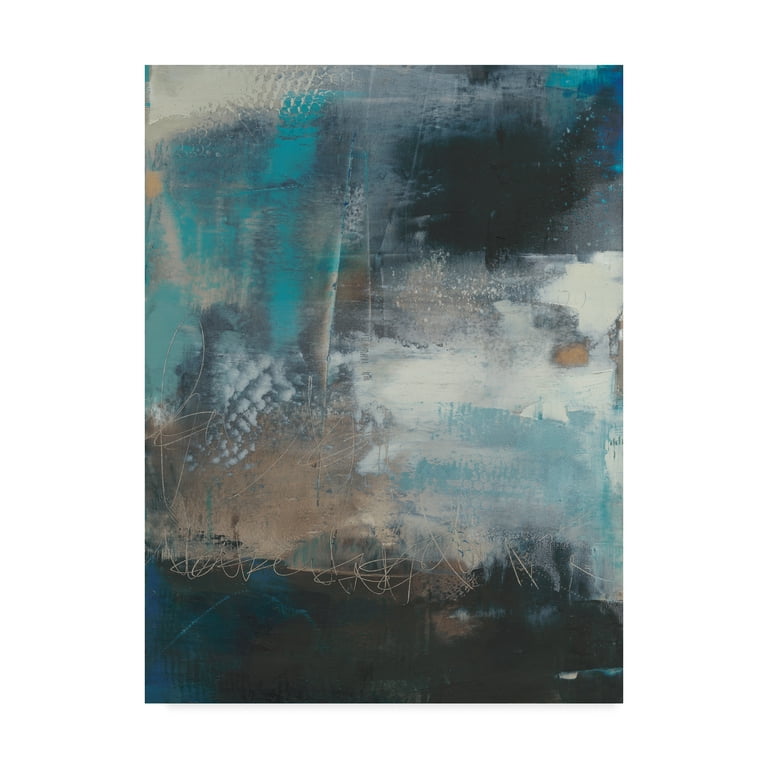This is a vertically aligned rectangular painting, likely on a canvas surface due to its textural appearance. The painting has no border and is surrounded by a solid white background, emphasizing its abstract nature. Starting at the bottom of the artwork, the predominant colors are black and brown, suggesting the ground. Above this, on the left side, there are intertwining brown lines, which might resemble curving shapes or elements of nature. To the right side, patches of blue and white add contrast.

Further up, a gray area appears, reminiscent of smoke, with two arm-like forms reaching upwards. These arms are shaded in gray with dark gray fingertips, and between them is a distinctly green arm with well-defined fingers, contributing to the abstract and interpretative nature of the painting. Additionally, there are cold brown and flat white areas around the center, with dark teal tints on the edges and blue accents that draw the eye. The top left corner features an off-white color interspersed with blue, blending into the overall abstract composition of the piece.